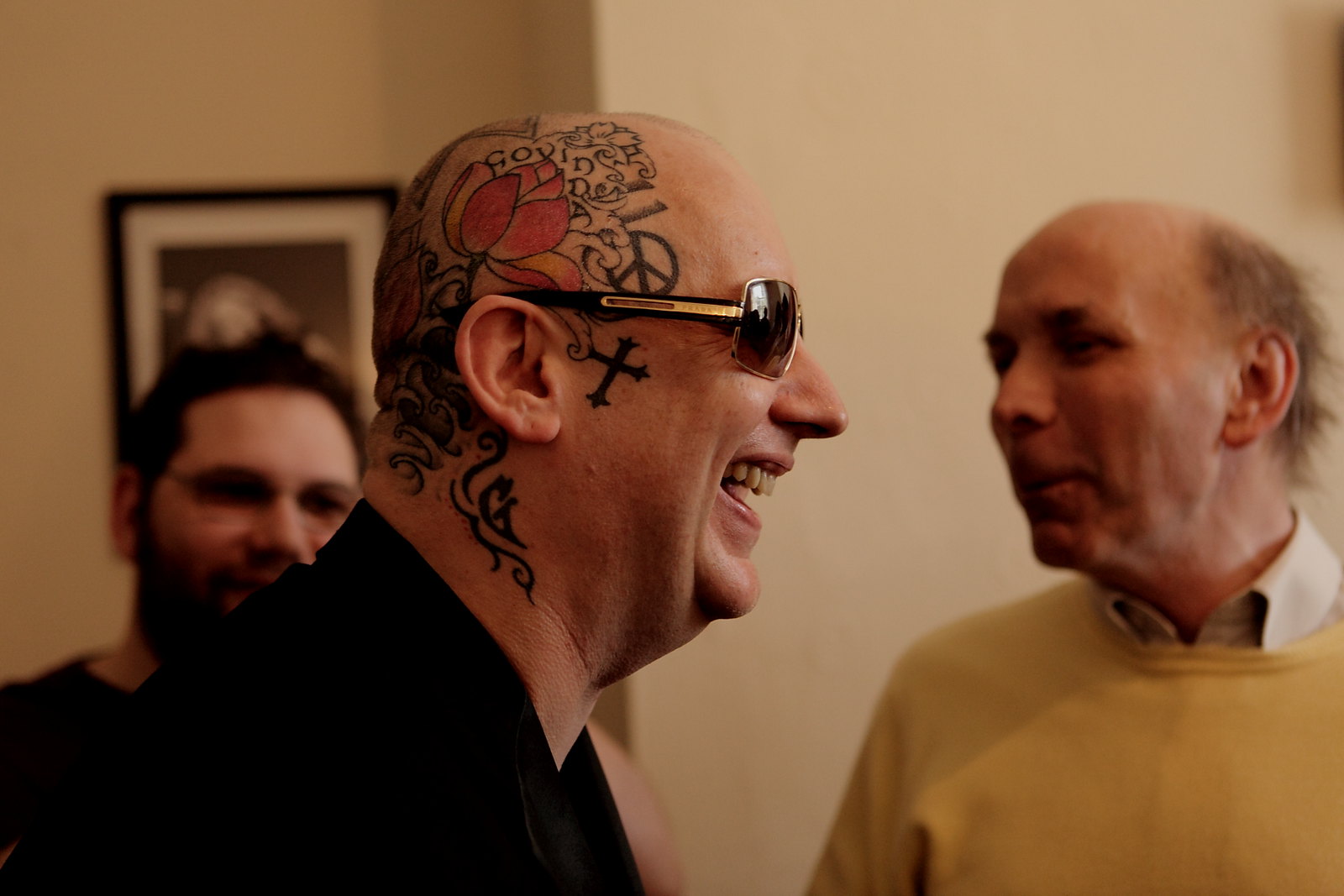The image captures three men standing indoors against a backdrop featuring a framed picture on the wall. The focal point is a bald, older man who appears side-profiled and smiling broadly, revealing a toothy grin. He's adorned in a black suit and distinctive black and gold sunglasses with dark red-tinted lenses. His head, devoid of hair, showcases an array of intricate tattoos, including a prominent red rose above his ear, a peace symbol, a gothic cross, the word "COVID," and various swirly designs that extend down his neck. To his right stands a balding, gray-haired man wearing a yellow sweater over a white undershirt, who gazes to the left of the frame. Behind Boy George, to his left, another man with dark hair and glasses stands in front of the wall art, contributing to the indoor ambiance of the scene.